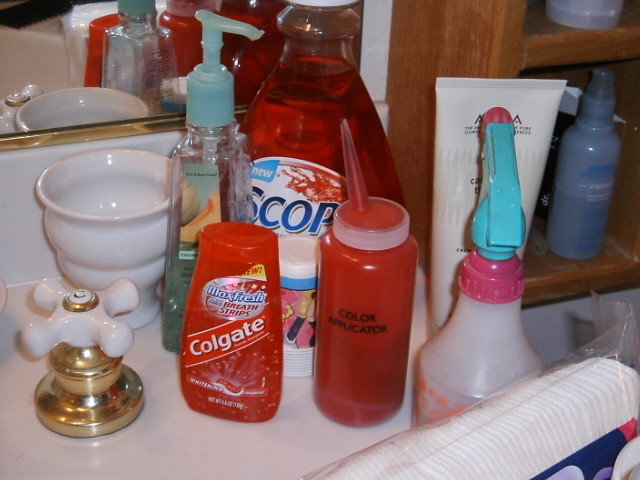On the bathroom sink, several products are meticulously arranged, suggesting a well-organized and perhaps upscale setting. The visible cold water knob is elegantly designed with a clean white finish and gold trim, indicative of a stylish decor. Among the items on the sink, there is a bottle of Scope mouthwash for fresh breath, a color applicator, and a container of Colgate breath strips. Additionally, there is an unidentified spray bottle, what appears to be Aveeno skin lotion, and a dispenser of hand soap. To the right of the sink, more shelves are packed with various products, though the specific items are not discernible in this view. A small bowl, resting near the hand soap, stands empty. The overall arrangement and quality of the bathroom hint at a sophisticated space, potentially used by an individual who values both functionality and aesthetics.